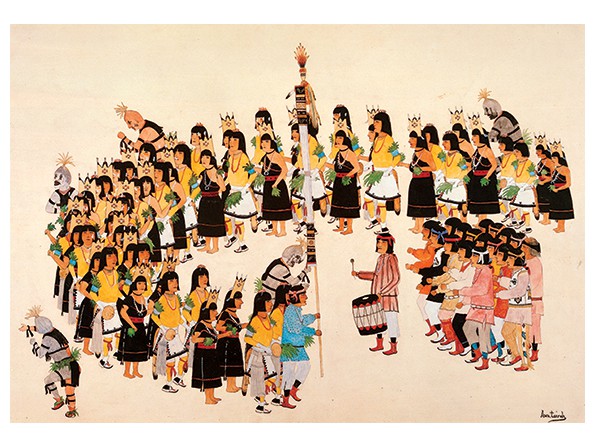The image depicts an old-world rectangular painting, approximately four inches wide and three inches high, with a light peachy-brown toned paper. The lower right-hand corner features an illegible artist's signature in black, speculated to start with an "A" and possibly ending with a "T". Dominating the painting is an ensemble of native people dressed uniformly. The women are adorned in black dresses with one-shoulder bare, accented by red sashes around their waists, short black bob hairstyles, and wooden three-pointed crowns. Their male counterparts wear white skirts paired with orange or yellow shirts, decorated with green leaves tied around their waists, blue armbands with yellow shirts, and some with grass accessories. 

Arranged in a semi-circle, about 40 individuals form a conga line, starting from the lower center and arcing back towards the left. On the right, a separate cluster of about 15 men seems to be dancing. This group includes figures with spiky hair resembling masks and gray-painted faces, heightening a sense of diversity within the assembly. Leading them is a drummer, marked by his distinctive attire: white pants, a long-sleeve red shirt, and a hat while holding a large drum and drumstick. An isolated dancer is also visible in the lower left corner. Adding an element of hierarchy or direction is a person holding a tall standard, white with black and gold accents, guiding the followers.